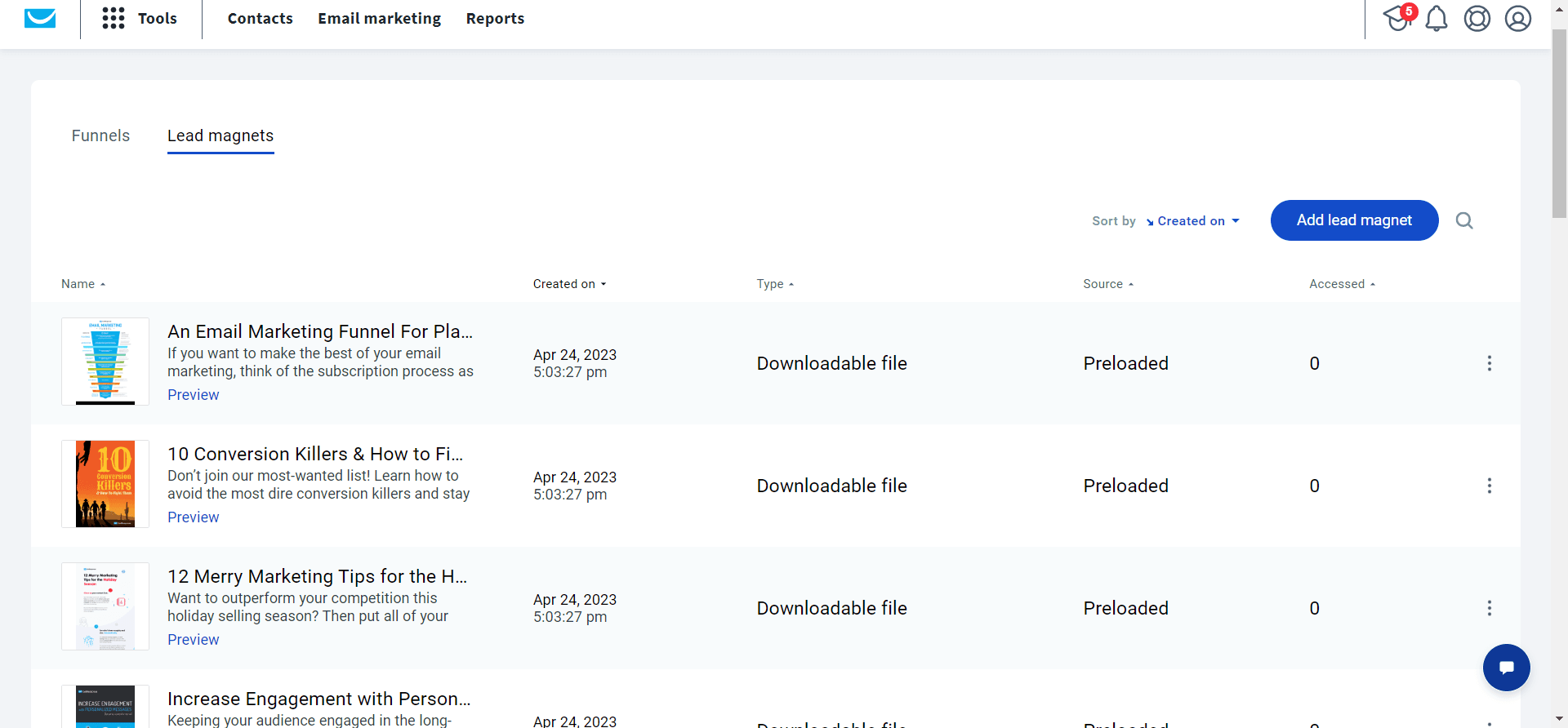This is a detailed screenshot of a webpage with a white background. In the upper left corner, there is a small blue envelope icon followed by a black line. Adjacent to it is an array of black dots with the label "Tools". Another black line follows, separating sections labeled "Contacts", "Email Marketing", and "Reports".

In the upper right corner, there are four icons: a graduation hat, a bell, a circle containing what appears to be a heart candy, and a circle with a human silhouette.

Below this upper toolbar, the webpage is bordered by a light gray margin. At the top left of the main white section, the word "Funnels" is displayed, followed by "Lead Magnets", which appears to be selected, indicated by a blue underline.

Beneath "Lead Magnets," four selections are listed. The first item is an "Email Marketing Funnel for PLA" with the description starting, "If you wanted to make the best of your email marketing think of the subscription process as..." This entry also notes it was created on April 24, 2023, at 5:03:27 PM, is available as a downloadable file, is pre-loaded, and currently, zero people have access to it.